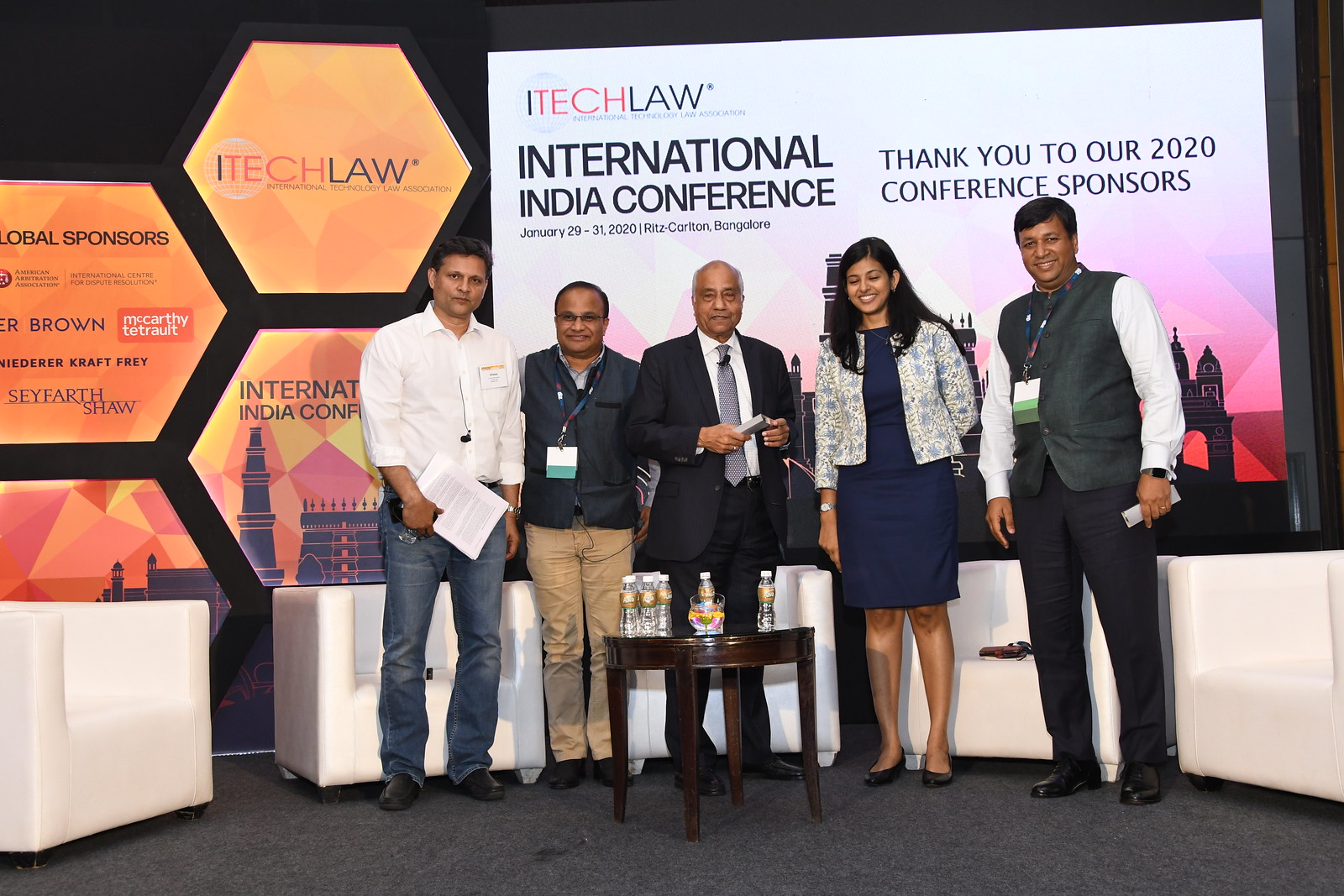This photograph captures a moment at the ITECH Law International India Conference held from January 29th to 31st, 2020, at the Ritz-Carlton in Bangalore. Five individuals—four men and one woman—are standing on an indoor stage, likely between conference sessions or during a photo shoot. Starting from the left, a man in a white shirt and jeans is holding a clipboard. Next to him is another man in khakis and a vest with a credential around his neck. The central figure is dressed formally in a suit and tie, while the woman, with her eyes closed, is wearing a blue dress. The man on the far right is also in a vest with credentials, paired with black pants. In front of them, a small table holds several water bottles, hinting at a refreshment setup. Behind the group are white sofas, and the backdrop features a black wall adorned with various posters. One prominent banner reads, "ITECH Law International India Conference," and acknowledges the 2020 conference sponsors, including some global sponsors such as Sefarth Shaw and McCarthy Tetrault. Hexagonal posters further decorate the background, adding to the conference ambiance.